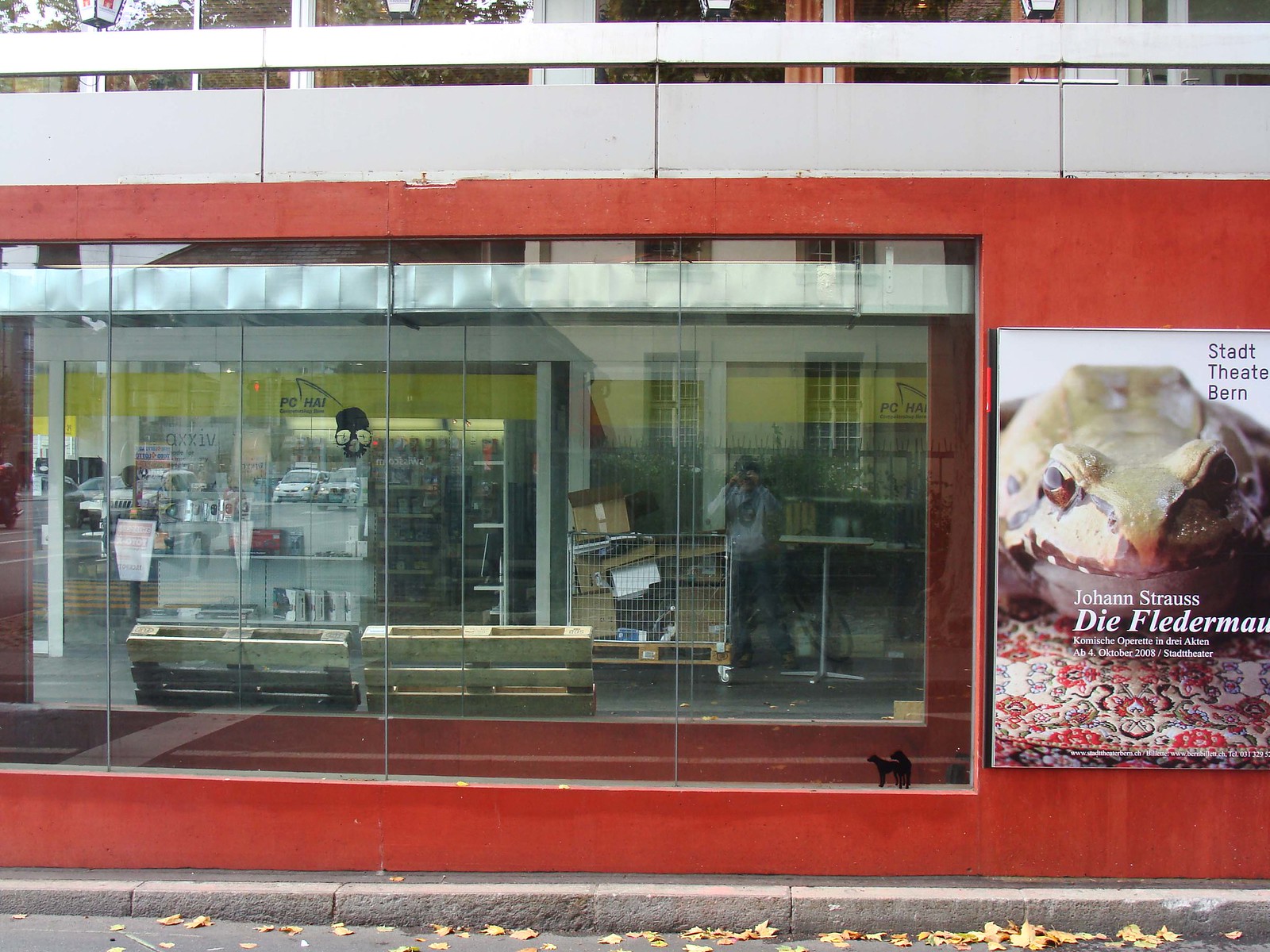This photograph captures the storefront of a building with a striking red exterior wall situated on a small sidewalk, with bricks separating it from the parking lot. A large glass window on the left side reveals the interior of the store, which appears to be under construction. Inside, racks are visible along with electronic equipment, boxes, and pallets leaning against the glass. A metal cart loaded with cardboard boxes is also present, and a man inside the store seems to be looking at the camera, possibly taking a picture.

To the right of the window, an advertisement featuring a frog sitting on an elaborate cushion is prominently displayed on the red wall. Despite the foreign language text, possibly German, the image of the frog is clear. Above the red wall, the building transitions to a white section with a small balcony railing and additional glass features on the second story.

On the concrete sidewalk below, a few orange leaves add a touch of natural color to the scene. The repeating panes of glass reflect the surrounding cityscape and also hold a curious statue of two black dogs intertwined together on the windowsill. This detailed view provides a comprehensive glimpse into the facade and ongoing activities within this under-construction storefront.